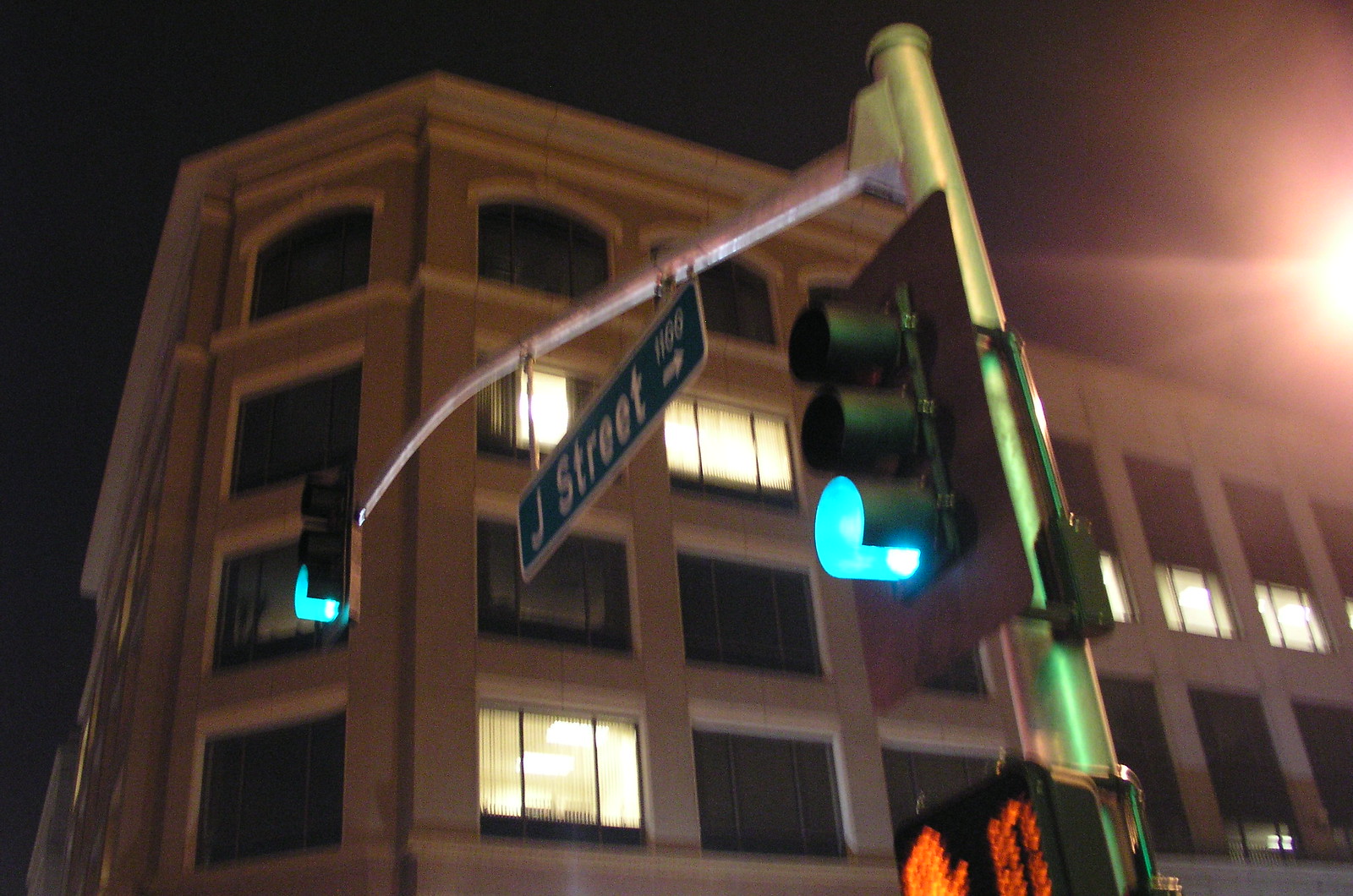In this nocturnal street scene, illuminated by unseen street lamps, we see a medium-height building in the background, likely an apartment or office building, with five floors. Several of its windows display lit rooms, particularly on the second, third, and fourth floors. Dominating the foreground is a traffic light mounted on a silver pole, glowing green to indicate smooth traffic flow. This pole features an arm extending into the street, holding a second green traffic light, appearing almost blue in the photograph. Suspended from the arm is a green street sign reading "J Street 1100" with a right-pointing white arrow. Additionally, a pedestrian signal beneath the traffic lights shows a red hand and a countdown timer indicating 10 seconds remain for crossing safety. Despite some motion blur, the image captures the urban essence of this nighttime setting.